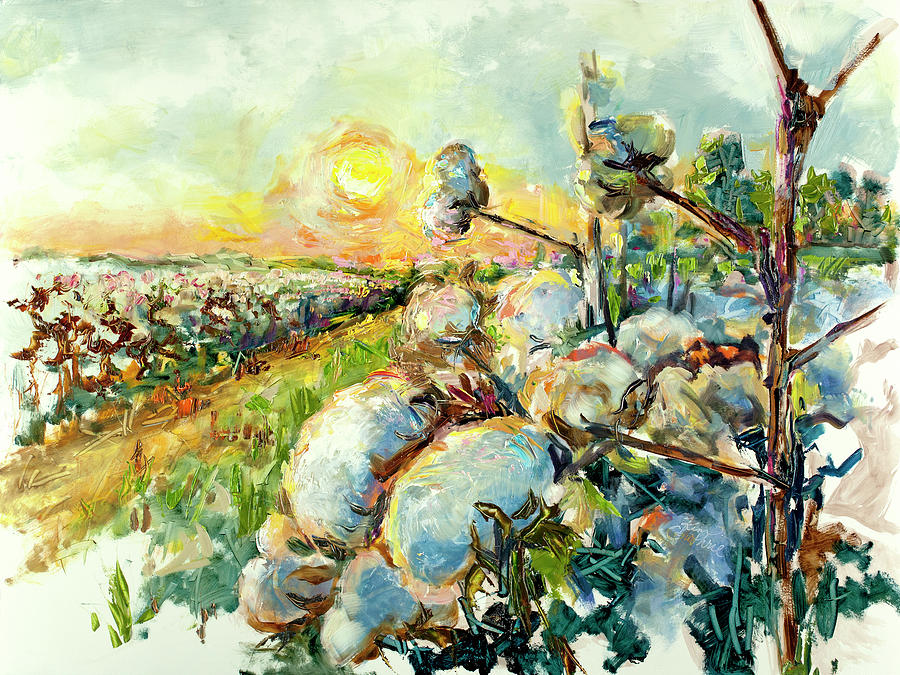This vibrant, romanticized painting showcases a sprawling cotton field under a colorful sunset. Dominating the right side of the image are cotton plants with brown twigs and white, fluffy cotton bulbs, framed by green leaves. In the foreground, a brown path edged with patches of grass meanders through the cotton field, leading into a valley on the left where more cotton plants grow abundantly. The sky is a spectacle of colors: a brilliant yellow sun with an orange border sits low on the horizon, casting a warm glow over the scene. Above it, the sky transitions through gradients of yellow, pink, and orange, blending into light blue, gray, and off-white clouds, evoking a serene summertime ambiance. The painting's use of acrylic or watercolor mediums, with its sketchy yet detailed style, adds a dynamic and expressive quality to this idyllic agricultural landscape.